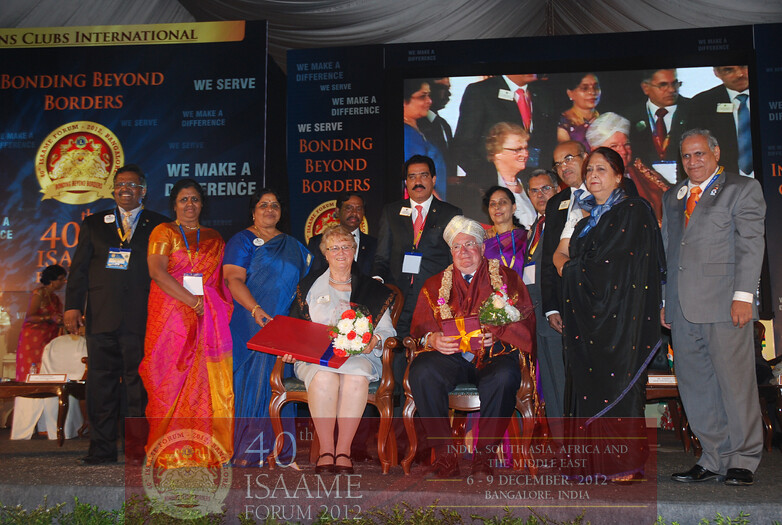This vibrant and joyful image captures a celebratory moment on a podium at a significant event in Bangalore, India. The stage is adorned with around twelve people, with the focal point being two elderly individuals seated in ornate wooden chairs at the center. The woman, holding a radiant bouquet of flowers and a large, beautifully wrapped red and blue gift, sits beside a man wearing a traditional Indian headdress and draped with a robe, who also holds a golden-wrapped gift and a similar bouquet. Smiles abound as they are flanked by ten others, including four women dressed in colorful, traditional Indian dresses and men in suits and ties, all seemingly honoring the seated couple. Behind them, a large video screen displays the phrase “Bonding Beyond Borders” multiple times, alongside other messages like "We Serve, We Make a Difference," hinting at the altruistic nature of the gathering. Prominently featured at the bottom of the image is a semi-transparent banner that reads: "40th ISAME Forum 2012, India, South Asia, Africa, and the Middle East, 6th through the 9th of December 2012, Bangalore, India," affirming the global and inclusive spirit of the event.